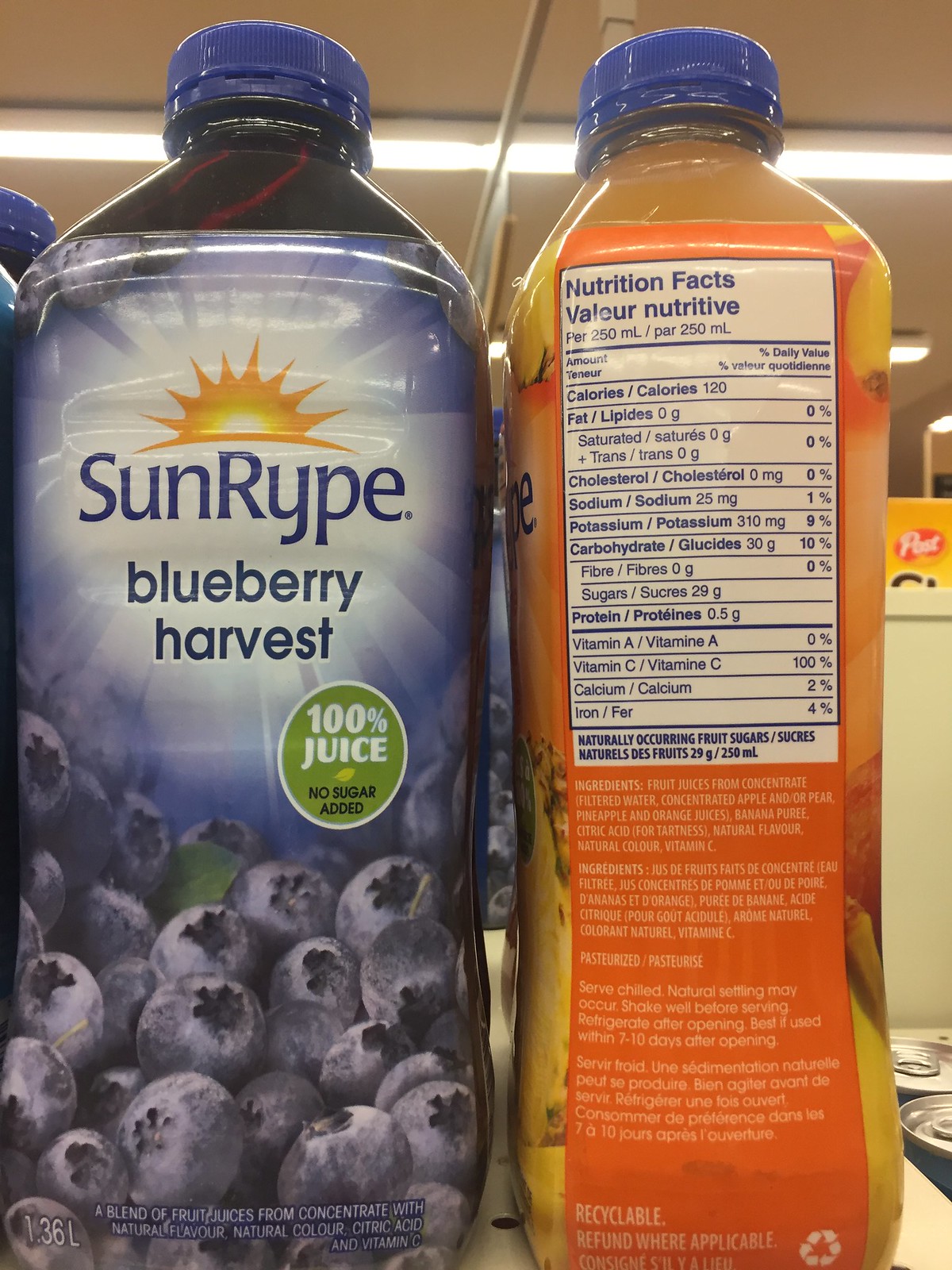In this image, we see two large bottles prominently displayed, occupying the entire frame. The bottle on the left features a blue lid and a visually striking label adorned with an array of artistically drawn blueberries at the bottom. The blueberries are depicted with intricate detail, showcasing the small black centers and light bluish-purple hues. The brand name "Sunripe" is prominently displayed above the label text "Blueberry Harvest." Just above the brand name, rays of the Sun are illustrated, symbolizing freshness and natural goodness. Additionally, within a green circular icon, the label proudly declares "100% Juice No Sugar Added."

To the right, we see the partial side view of another juice bottle with an orange background. The label on this bottle displays the nutrition facts in white text, which is intricately detailed albeit quite small. Beneath the nutrition facts, the label also bears the word "Recyclable" printed along the bottom edge, emphasizing the brand's commitment to sustainability. The bright orange background of this bottle contrasts vividly with the more subdued blue and green tones of the bottle on the left, creating a dynamic and visually appealing composition.